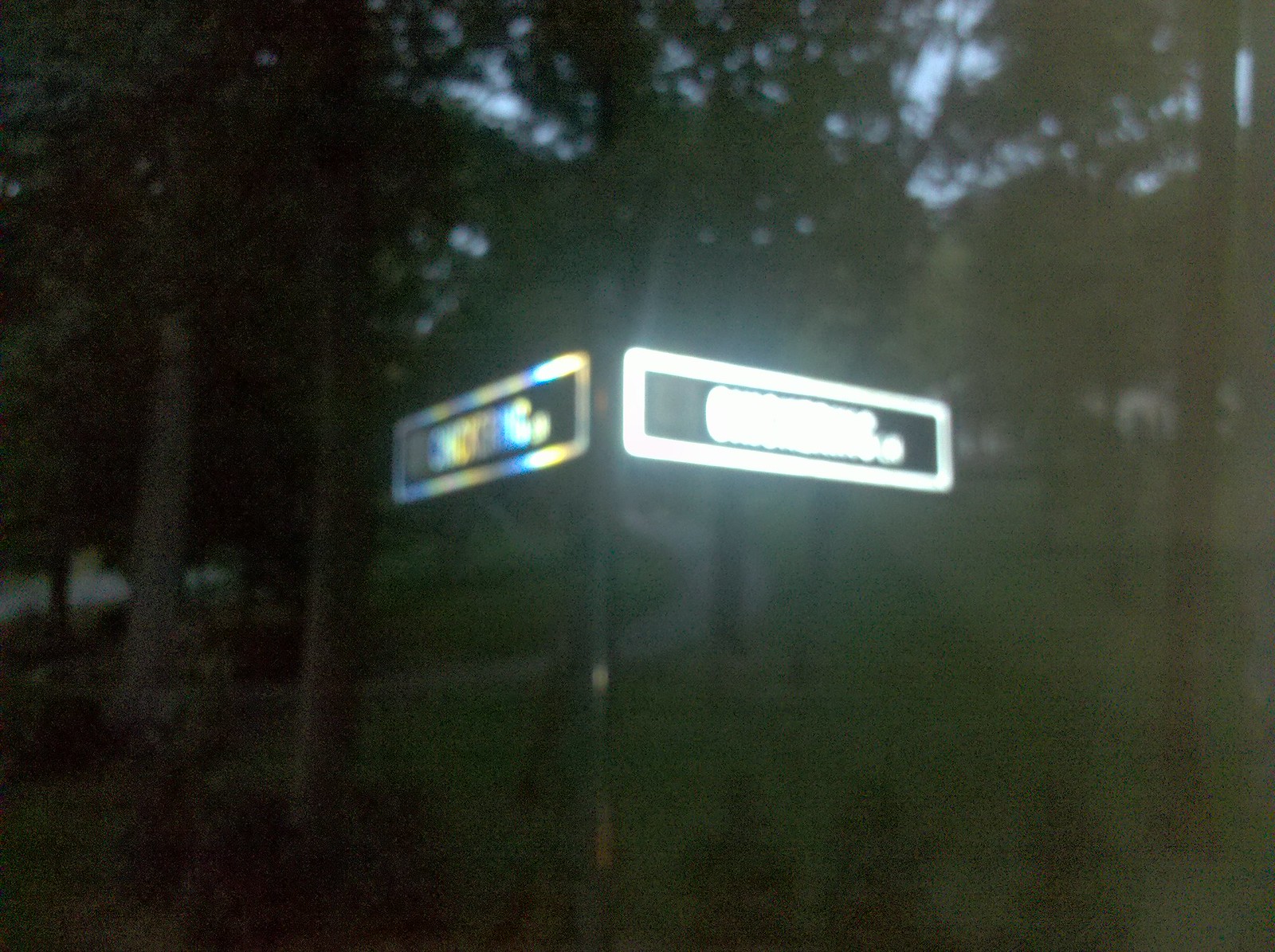The photograph captures a nighttime scene at what appears to be a park or pathway intersection. A walking trail curves into the distance at the center of the image, flanked by trees and short plants. Prominently featured are two metal street signs mounted on a green pole, arranged in a V-shape, pointing in opposite directions to mark the corner of intersecting paths. Due to glare from reflective gloss and the camera’s bright white light, the text on the signs is illegible, though one appears to start with the letter "C." The scene is dimly lit, with the glowing signs standing out against the darkening environment, where tall trees and some grass are discernible in the background. The picture conveys a sense of quiet and seclusion typical of a park at dusk or night.